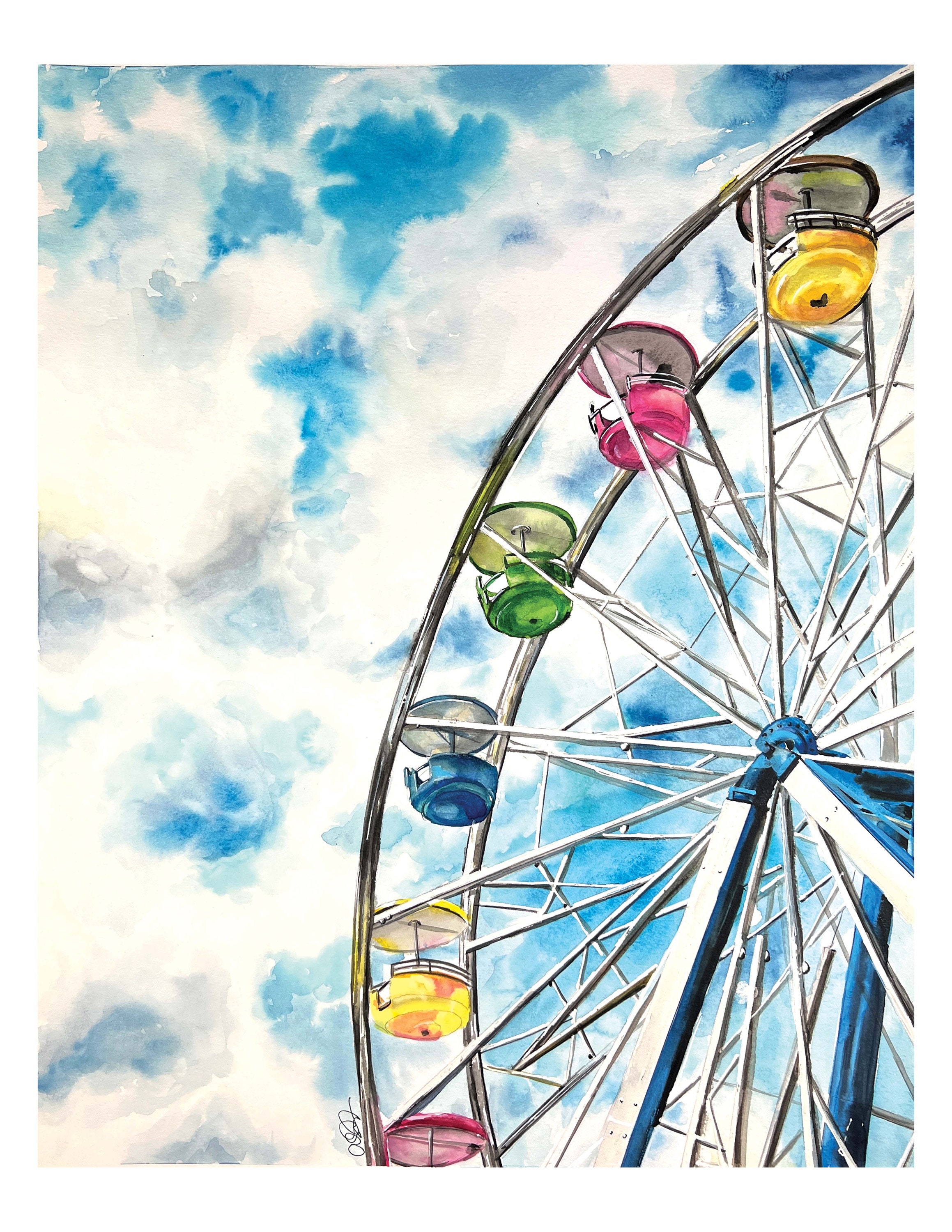This artistic watercolor painting vividly captures a portion of a classic ferris wheel. The wheel itself features a white, spoked design with gray railings adorning its outer edge. At the core of the structure is a blue center hub, from which blue and white pillars extend outward, adding to the intricate details of the ferris wheel's anatomy. Suspended from the structure are charming, old-fashioned cars in the shape of teacups, each topped with a sun umbrella—reminiscent of a bygone era. The cars are painted in a palette of pastel and bright colors, including pink, yellow, blue, and green, though the scene appears devoid of any riders. The backdrop is a dramatic sky, painted with heavy strokes of white and gray to depict cloud cover, contrasted against a deep blue background, enhancing the nostalgic and serene atmosphere of the scene.